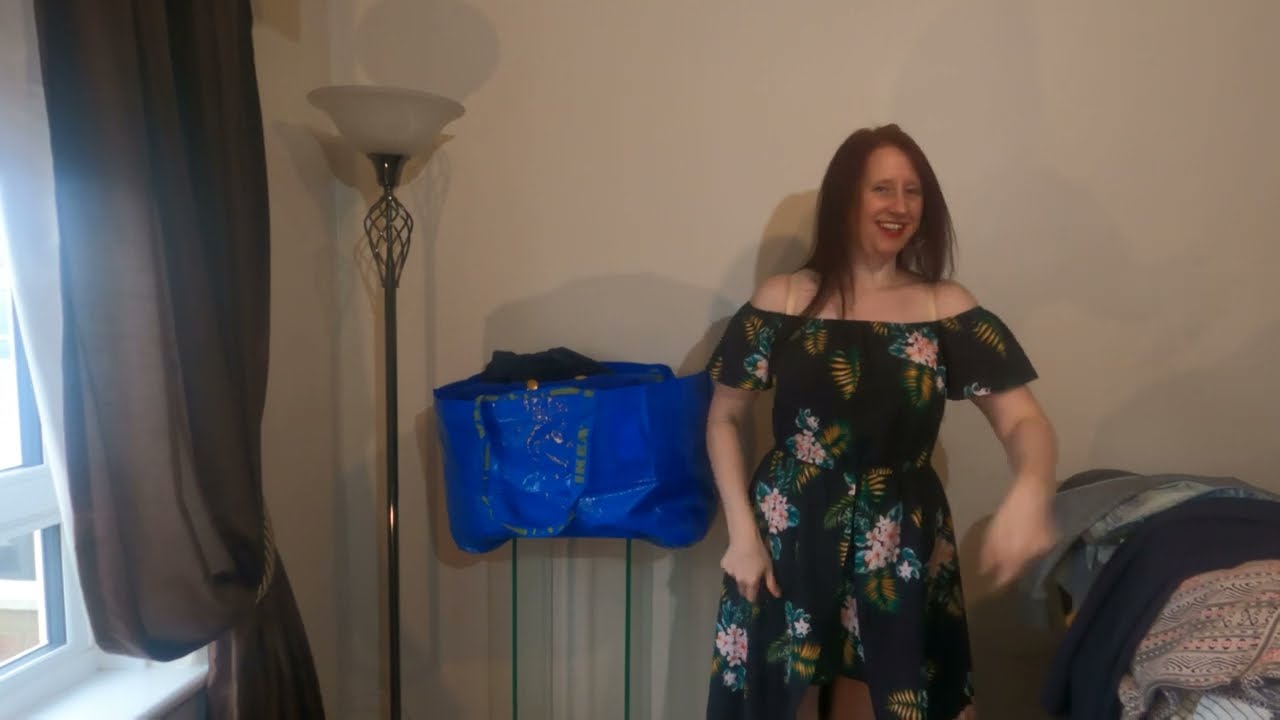In a low-quality, slightly blurry photograph, a middle-aged white woman stands inside a dimly-lit room. She is right of center, wearing a strapless black dress adorned with floral patterns that leave her shoulders bare. Her long, straight dark brown hair extends a little past her shoulders, and she smiles warmly at the viewer, showcasing her teeth and wearing red lipstick. To her left, there is a black reusable shopping bag resting on what seems to be a radiator or stand, blending somewhat into the backdrop of a beige or tan-colored wall. Further to the left, a decorative vertical lamp stands beside an open window draped with brown curtains. To the right of the woman, there is a pile of knitted blankets or clothes, possibly on a couch, completing the scene.